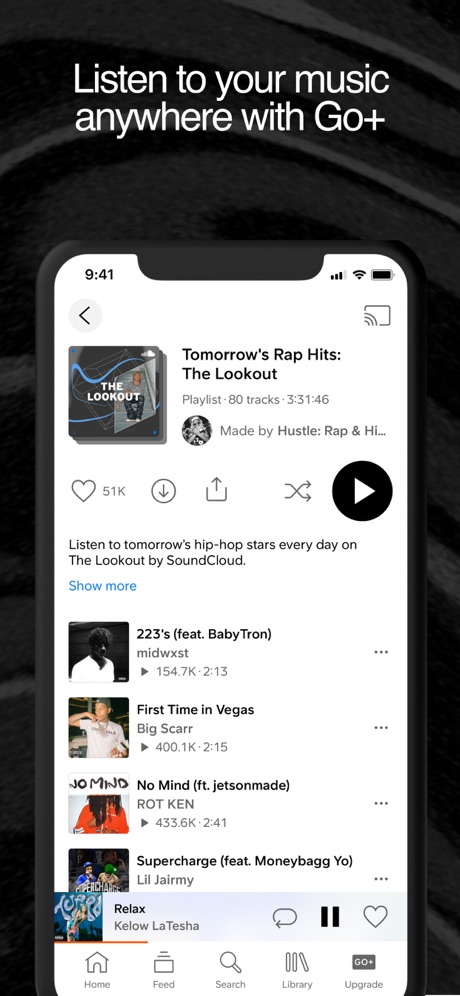This image features an advertisement shaped like a smartphone, set against a black background with swirling patterns. The central focus is a depiction of a phone screen displaying a music streaming app. Above the phone image, bold text reads, "Listen to your music anywhere with Go+," with the "+" symbol accentuating the message.

On the phone screen, the time is set to 9:41, and the battery is fully charged. At the top, the current playlist is titled "Tomorrow's Rap Hits" by The Lookabout. The playlist cover is prominently displayed, showing details that it contains 80 tracks, with a total duration of 3 hours, 31 minutes, and 46 seconds. Created by Hustle Rap and another contributor, it boasts 51,000 likes. Users have the option to download or play the tracks directly.

The advertisement prominently encourages listeners, "Listen to tomorrow's hip-hop stars every day on The Lookout by SoundCloud." Beneath this slogan, there is a "Show More" option that reveals additional albums available for listening. The highlighted albums include:
- "223's," featuring Babytron and Midwest
- "First Time in Vegas" by Big Scar
- "Yo Mind" (or "Joe Mind, No Mind") by Jetson Made and Rotkin

This visually rich and engaging ad targets rap enthusiasts, inviting them to explore and enjoy a curated selection of emerging hip-hop tracks.